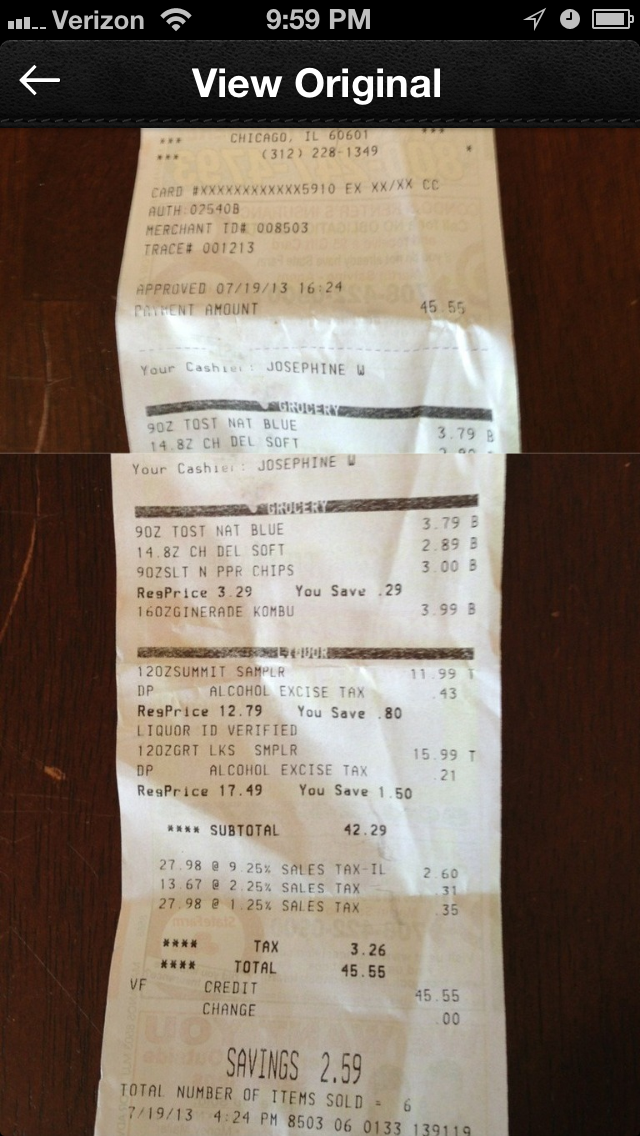The color photograph depicts two images of receipts displayed on a phone interface against a brown wood background. At the top of the image, the phone status bar, showing Verizon, the time (9:59 p.m.), and various status icons, frames the scene. Below this, to the left, are a left-facing arrow and the text "View Original" in a black band, indicating navigational elements of the phone interface.

The receipts, white paper with black print, dominate the image. The upper receipt occupies the top third of the picture, detailing a grocery transaction with a subtotal of $42.29, a total amount of $45.55, and a savings of $2.59. The cashier's name, Josephine, and the date, 7-19-13, are prominently displayed. The lower receipt, seemingly a continuation or another segment of the same transaction, extends across the bottom two-thirds of the image, reinforcing the total amount of $45.55 paid and including cashier Josephine's name again.